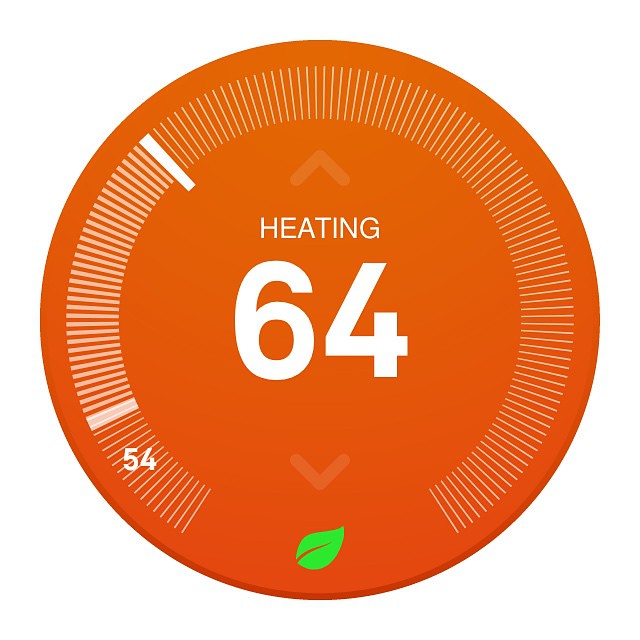A detailed digital interface display of an HVAC (heating, ventilation, and air conditioning) system is shown. At the center of the display is an orange circular zone, which is brighter at the top than at the bottom. Within this circle, "HEATING" is prominently displayed in capital letters. Beneath this label, the number "64" is shown in large, bold white numerals, indicating the current temperature setting.

Subtle arrows are positioned above and below these characters, suggesting options for adjusting the temperature. Directly below the temperature readout, a small green leaf icon is visible, potentially denoting an eco-friendly or efficiency mode.

Encircling the orange center, a pattern of white dashed lines creates a ring, marking temperature increments. On the lower left side of the ring, the number "54" is marked along the dashed lines. Above this, a thicker section of dashed lines appears, indicating a specific range or setting. This thick dashed section is followed by a narrow gap before a solid, thick white line segment. Beyond this thick line, the dashed lines resume their thinner appearance, continuing around the circle.